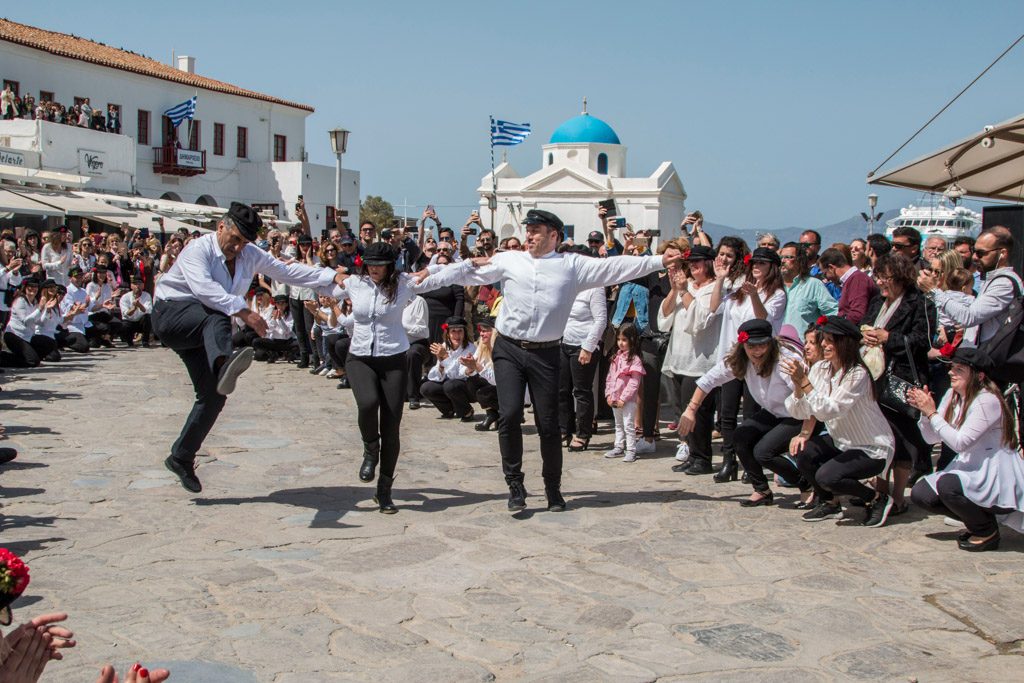The image captures a lively outdoor scene with a crowd gathering on a gray cobblestone area, surrounded by clear blue skies and faint mountain ranges in the distant background. Dominating the background is a white building capped with a small blue dome, next to which flies a blue and white flag that closely resembles the flag of Israel. Another flag with blue and white stripes and a white cross on the top left corner is also visible on a building to the left. Central to the scene, three dancers—two males flanking a female—all dressed in black pants, white shirts, and black caps, are energetically performing, with the man on the left raising one leg high into the air and the other man extending a hand toward the woman in the middle. Their dance is a focal point for the approximately 75-80 spectators forming a circle around them, many of whom are clapping and dressed in similarly coordinated outfits, contributing to the festive, communal atmosphere. Some onlookers can be seen cheering from a balcony, adding to the overall sense of joy and celebration.